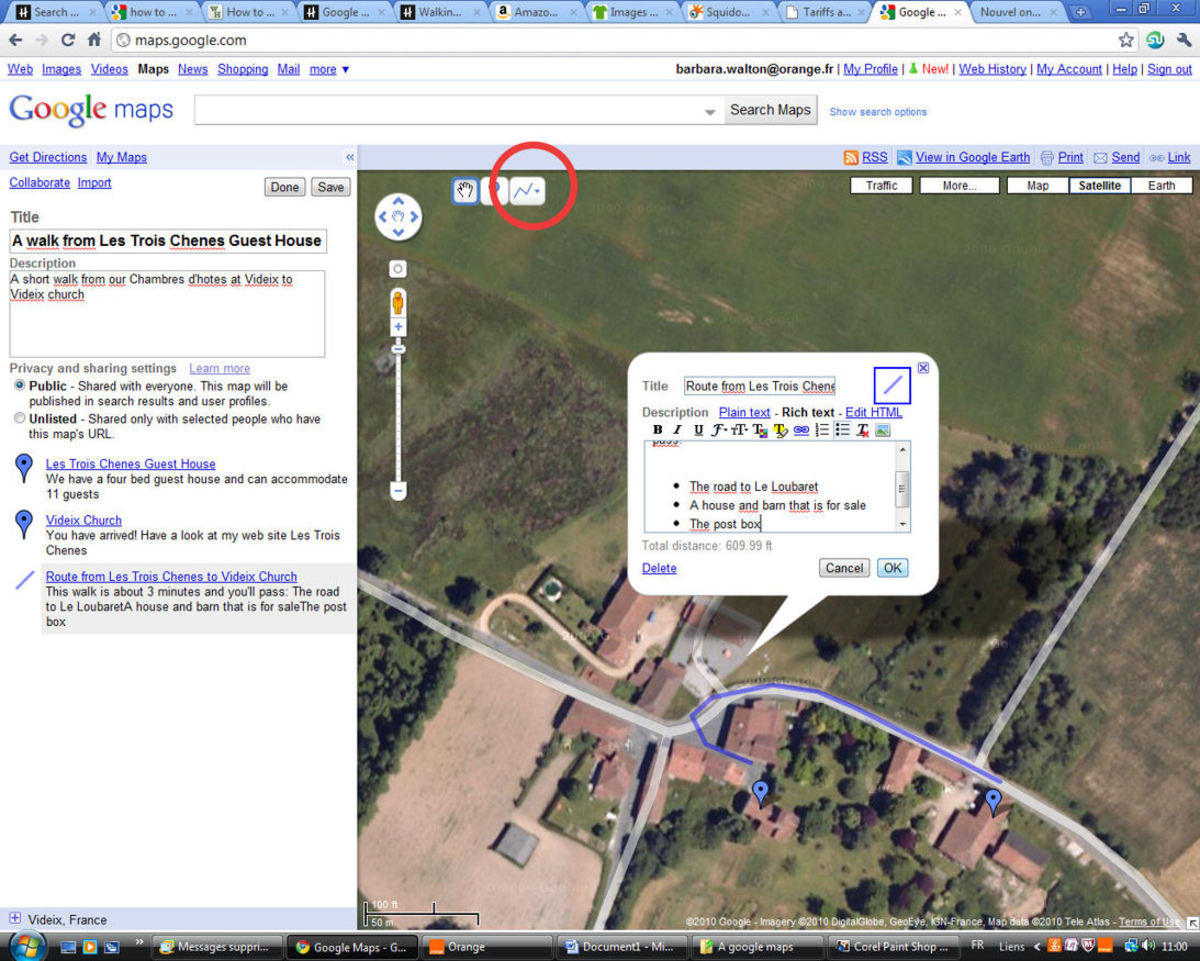**Caption: A Scenic Walk from Les Trois Chênes Guest House to Videx Church**

This detailed Google Maps image illustrates a short but picturesque walk from Les Trois Chênes Guest House to Videx Church. The route, marked by a distinctive blue line, starts at Les Trois Chênes (translated as "The Three Oaks" in French) and guides you through verdant green fields and lush trees, with patches of brown earth visible from an aerial perspective.

The guest house, located in a charming rural area, boasts four comfortable bedrooms and can accommodate up to 11 guests. As the route unfolds, it leads directly to the quaint and historic Videx Church, a peaceful landmark in the vicinity.

At the bottom of the map, options for privacy and sharing settings are visible, with this particular map marked as "Public," meaning it can be found in search results and user profiles. For those eager to explore this beautiful walk themselves, further details and the route can be viewed on the guest house's dedicated website.